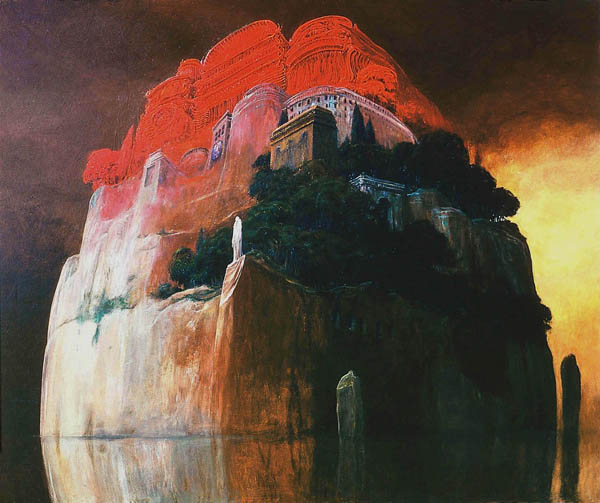The painting depicts a dark and ominous scene with a large, rocky formation reminiscent of a towering cliff or mountaintop, almost apple-shaped. Perched precariously atop the stone is a castle-like structure made of grey stone, blending seamlessly with the rocky base. The castle, featuring several towers with pointed roofs, occupies nearly the entire cliff, leaving little to no overhang. Adding to the eerie atmosphere, the sky above is overcast with swirling clouds, casting a gloomy pall over the scene.

To the right of the stone formation, dark hues suggest dense shrubbery or possibly trees, contributing to the overall darkness of the image. Above the central building, an additional structure or extension is rendered in orange and red tones, standing out starkly against the otherwise monochromatic palette.

The background features a gradient of colors, from dark brown at the top to an almost fiery yellow and orange on the bottom right, hinting at a source of light or fire. Reflections in the water at the base of the cliff show the silhouette of the stone and the castle, with small waves crashing onto the rocky foundation, enhancing the desolate and mysterious mood of the painting.